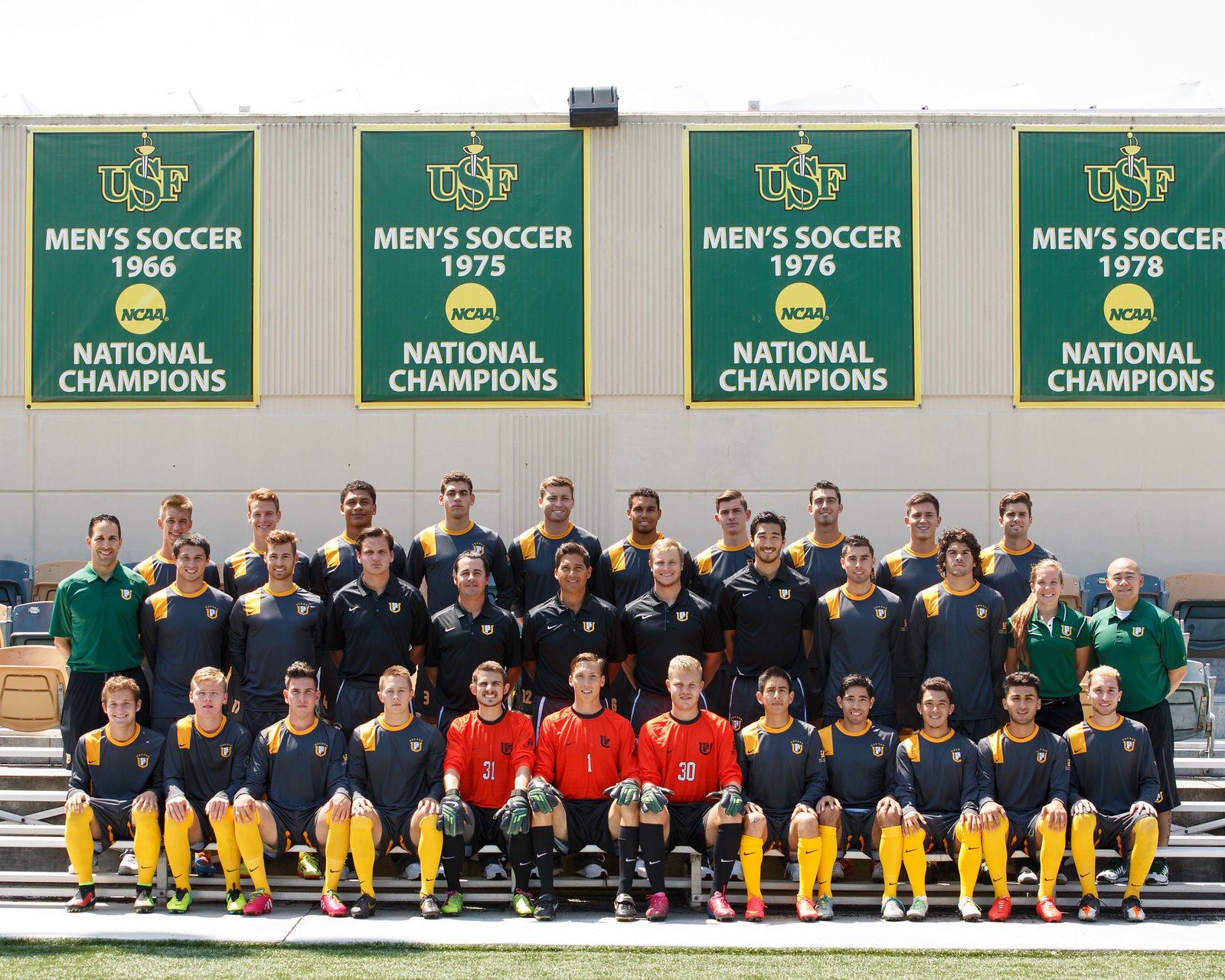This is a detailed, wide rectangular photograph of the University of San Francisco (USF) men's soccer team, posed on bleachers. The team is arranged in three rows: the front row is sitting with hands on knees, the middle row of medium-sized players is standing, and the back row of taller players also stands with hands behind their backs. Most team members wear navy blue jerseys with yellow accents and bright yellow socks, sporting various colored cleats. The goalkeepers, positioned in the middle of the front row, are distinguished by their red jerseys with black collars. The group includes three coaches in green short-sleeved shirts with collars—two males and one female. Positioned against a white building, possibly a gymnasium, the backdrop showcases four vertical green banners with yellow borders that celebrate USF’s national championships from 1966, 1975, 1976, and 1978. Each banner has "USF Men's Soccer" in green font with yellow outlines at the top.